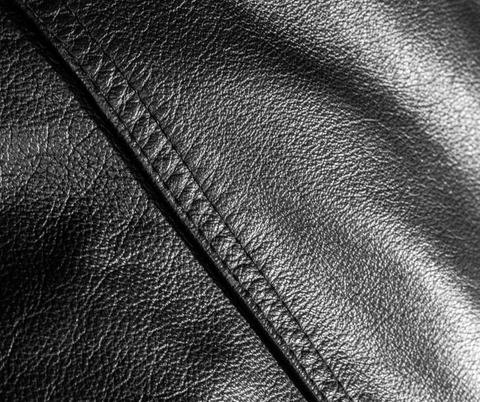The image depicts a close-up of a piece of black leather, likely part of a high-quality garment such as a jacket or pants. The leather has a fine grain with natural craggly and jagged lines, indicating its authenticity as an animal product. It has been well-maintained, potentially treated with oil to enhance its glossy appearance without leaving a greasy residue. The leather is illuminated by light, creating a shine that highlights its rich, dark color. A prominent feature in the image is a seam, specifically a double-seam stitch, with a raised flap showcasing the meticulous and uniform stitching. The fine, tight stitches suggest that a professional meticulously crafted the garment, emphasizing its luxurious and likely expensive nature.